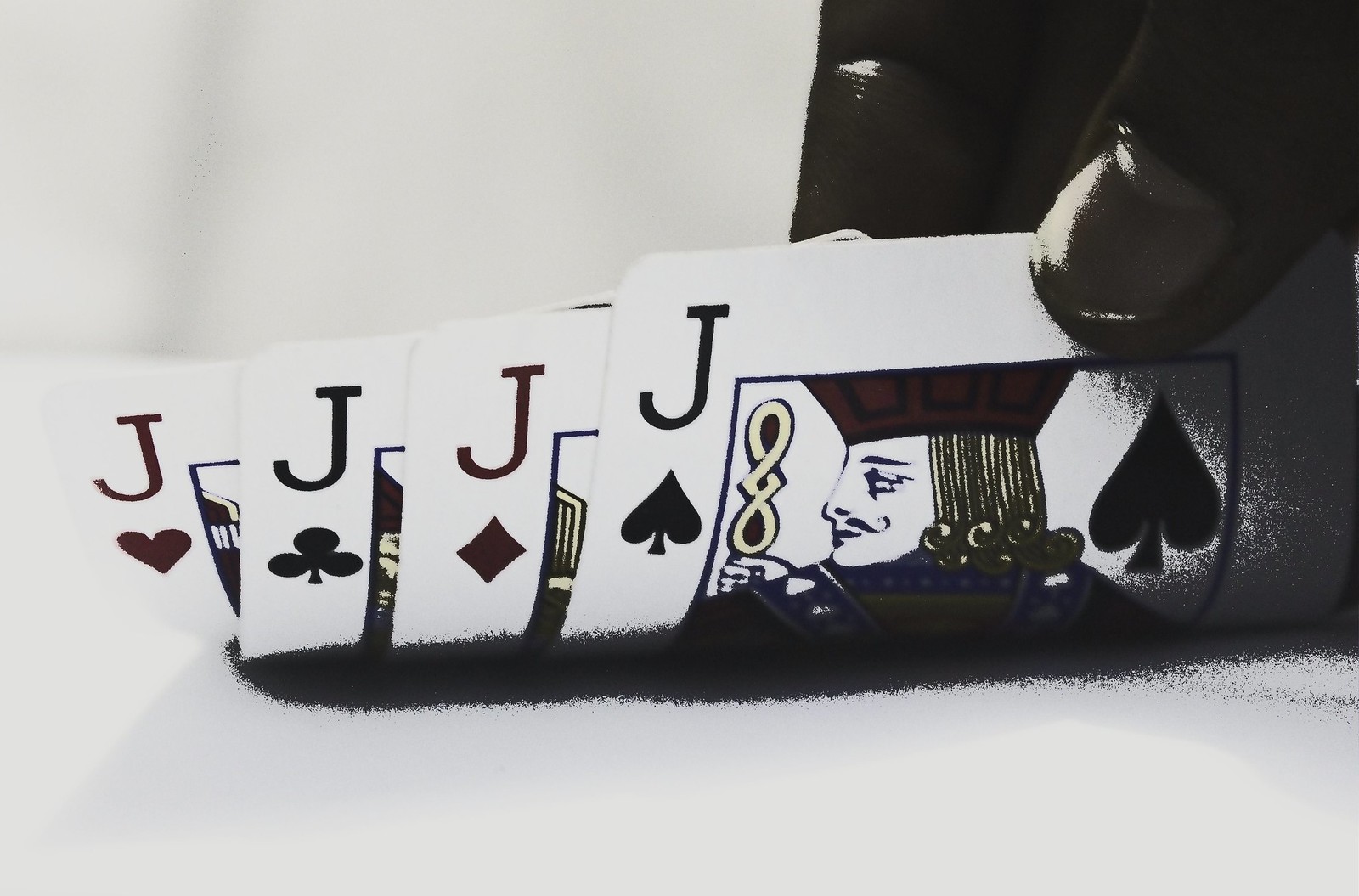In a slightly overexposed photograph, a player reveals four cards during a card game. The cards, partially arced upwards under the player's thumb, are all lying flat on a white table with a subtle shadow creating a blurred effect underneath. The cards, identified as standard Bicycle playing cards, consist of the jack of hearts, the jack of clubs, the jack of diamonds, and the jack of spades, all facing left. The prominence of their bright designs stands out against the stark white background. Despite the overexposure, the vibrant details are discernible: the red of the jack of hearts and diamonds, the blue ornate detailing on the jack of hearts' attire, the red in his hat, and the gold in his hair. The player's thumb, positioned on the upper right of the image, is almost completely shrouded in shadow, adding a dramatic contrast to the otherwise minimalistic scene.